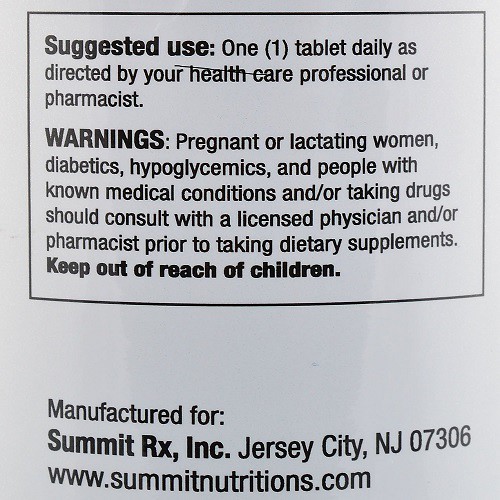The close-up image depicts a detailed warning label on the back of a dietary supplement or drug product set against a white background. The label features a thin black border around the top portion, delineating a box. It begins with "Suggested Use" in bold, followed by instructions advising users to take one tablet daily as directed by a healthcare professional or pharmacist. The label then presents "Warnings" in bold, indicating that pregnant or lactating women, diabetics, hypoglycemics, and individuals with known medical conditions or those taking medications should consult with a licensed physician or pharmacist prior to use. It emphasizes in bold "Keep out of reach of children." At the bottom, the label specifies, "Manufactured for Summit Rx Inc., Jersey City, New Jersey 07306," alongside the website, www.SummitNutritions.com.